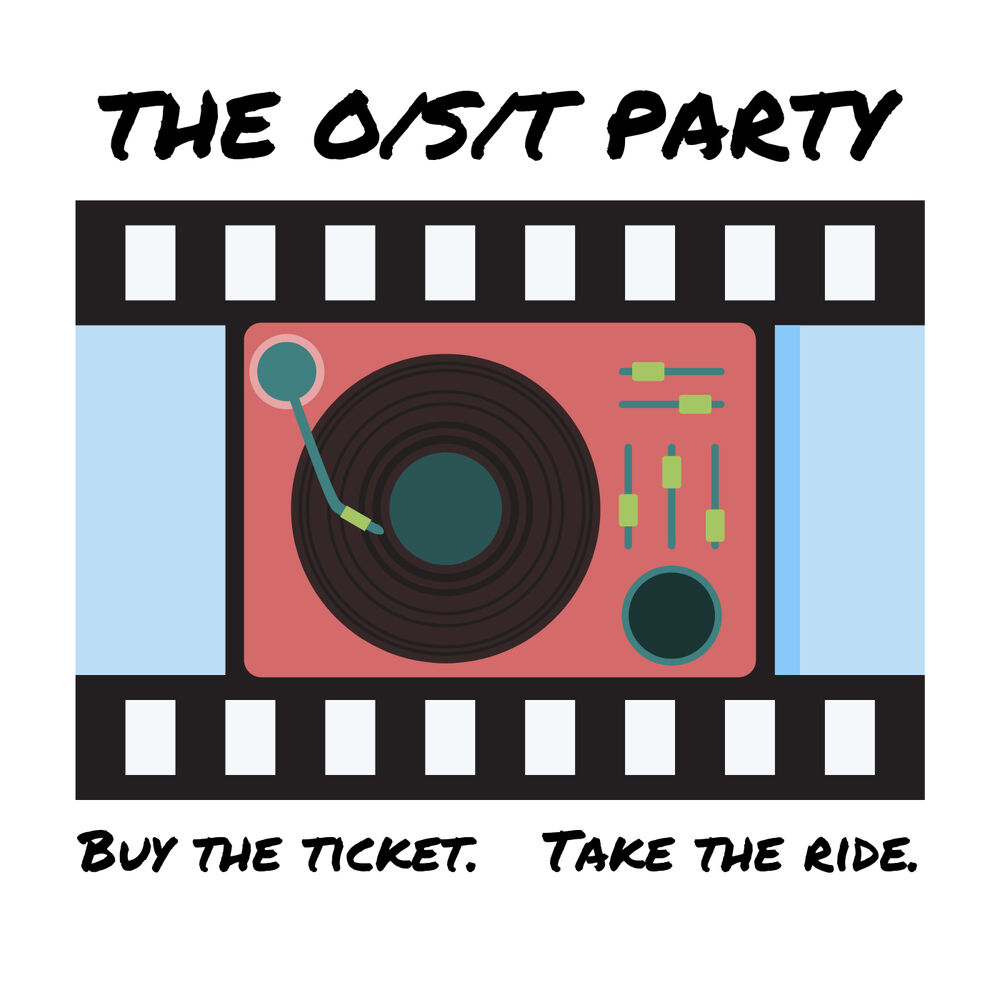This advertisement image features a vintage-inspired design with a prominent film strip motif at the top and bottom. At the very top, in bold black letters, the text reads "The OSIT Party." Directly below this header, the film strip element is depicted with black edges and white steps, reminiscent of old-time cinema reels. The central focus of the image is a rectangular, red and orange DJ record player, set against a contrasting blue background. On the left side of the player, there is a blackish-brown circle resembling a vinyl record, with a green inner circle indicating the record's label. The record player includes green knobs, likely for adjusting sound settings such as the bass, treble, and volume. Below this central image, another film strip spans the width of the advertisement. At the bottom, the phrase "Buy the ticket, take the ride" is prominently displayed, encouraging engagement and participation.